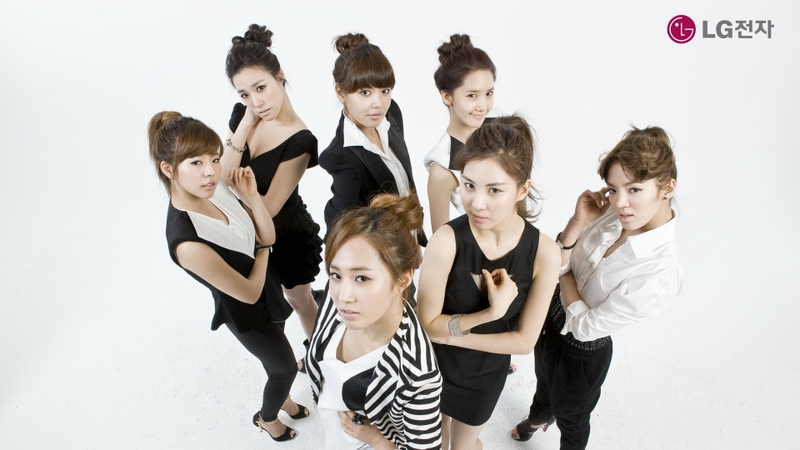This image appears to be an advertisement for the LG brand. In the upper right corner, there's LG’s signature purplish-red circular logo, accompanied by the letters "LG" in gray type, followed by Korean characters that likely spell out "LG." The scene captures seven young Asian women, potentially in their twenties, dressed in various combinations of black and white attire. Some are wearing black dresses, others sport black pants with white long-sleeved collared shirts or a black and white striped shirt. Their outfits are completed with matching professional hairstyles, many opting for buns. The angle of the shot is slightly elevated, making the women look up towards the camera, their expressions ranging from subtle smiles to professional, sultry looks. The background is predominantly white with a slight gray tint. The overall composition and color scheme reflect a modern, cohesive, and stylish aesthetic, strongly indicating this is a promotional image for LG.